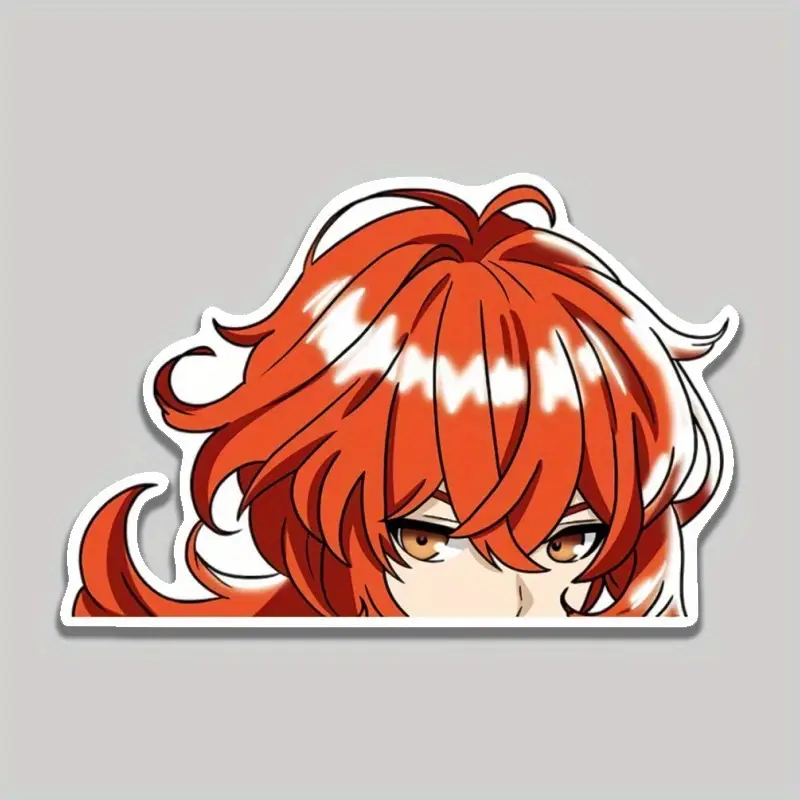The image showcases a 3D animated depiction of a woman with voluminous, flowing ginger hair and amber eyes. Set against a plain light gray background, the partial headshot captures her from the base of the nose to the top of the head. Her hair, characterized by dynamic bangs and locks sweeping in various directions, especially to the left, gives a sense of movement. The details focus on her pale skin and expressive eyes, which gaze downwards toward the bottom left of the image. The cutout is shaped to match the contours of her hair, suggesting it might be a sticker or a prototype for a print. The sticker itself has a white border that contrasts sharply with the gray backdrop, enhancing the vividness of the character's orange tones.